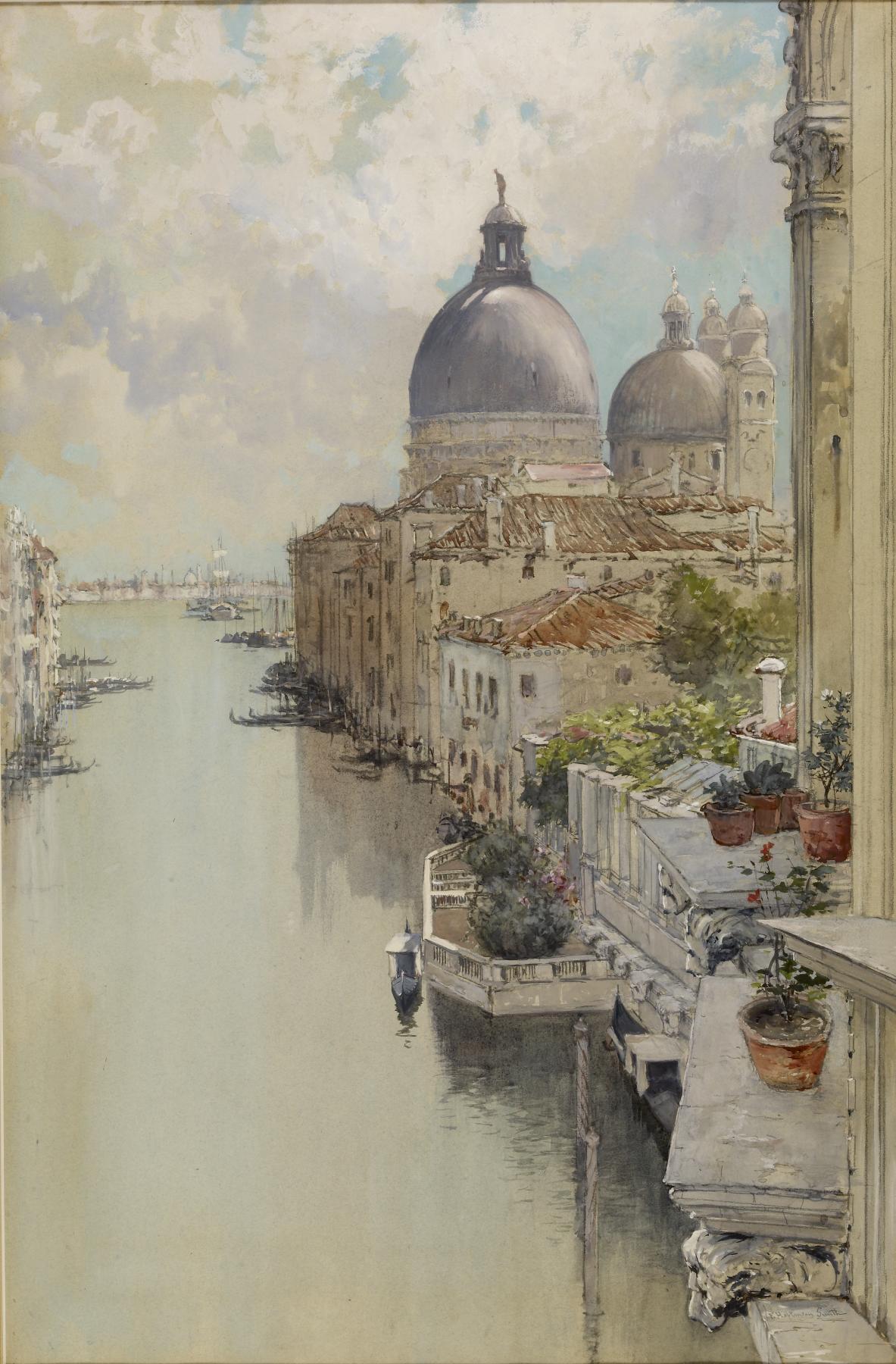This painting vividly depicts a picturesque canal scene, reminiscent of Venice, with lifelike details and a serene, almost whimsical atmosphere. Dominating the view are numerous buildings lined up along the right bank of a bluish-green canal, seen as if we are leaning out of a nearby window. The buildings immediately in sight feature small ledges outside open windows, adorned with various potted plants—one ledge with a single pot, another with four, and yet another closer to the water showcasing three pots. 

Further down the canal, the architecture alternates in height and style, with some structures exhibiting roofs in disrepair, while others proudly display their silvery-gray domes, possibly part of a grand church or historic building, reflecting the rich cultural heritage of the area. On the right, some balconies overlook the tranquil, still water of the canal, which hints at leading out to a larger body of water, such as a bay or the sea.

Several boats are moored next to the buildings, emphasizing the calm, unhurried pace of life. A sparkling light in the water adds a touch of enchantment to the scene. In the far background and to the left, more white buildings come into view, adding depth and dimension to the landscape. Above, the sky is a mix of blue with hints of white, gray, and even a touch of green, creating a captivating, almost dreamy ambiance that completes this stunning piece of art.